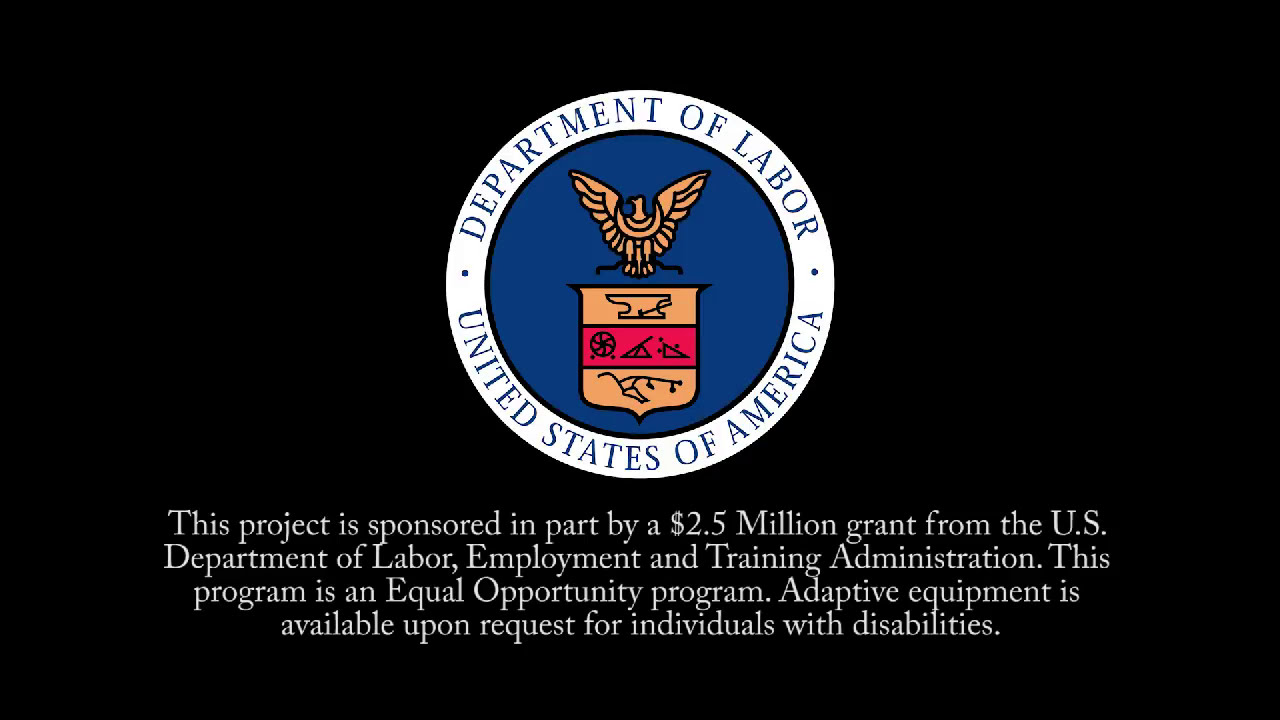The image features a black background with the emblem of the U.S. Department of Labor prominently displayed in the center. The emblem is a circular logo with a white outer border and a blue inner circle. At the top of the white border, in blue text, it reads "Department of Labor," and at the bottom, it reads "United States of America," separated by two small dots. In the center of the blue circle, there is a gold eagle above a crest that has three sections: the top section is gold with a symbol, the middle is a red stripe with additional symbols, and the bottom is gold with more symbols. Below the emblem, there is white text stating: "This project is sponsored in part by a $2.5 million grant from the U.S. Department of Labor Employment and Training Administration. This program is an equal opportunity program. Adaptive equipment is available upon request for individuals with disabilities."